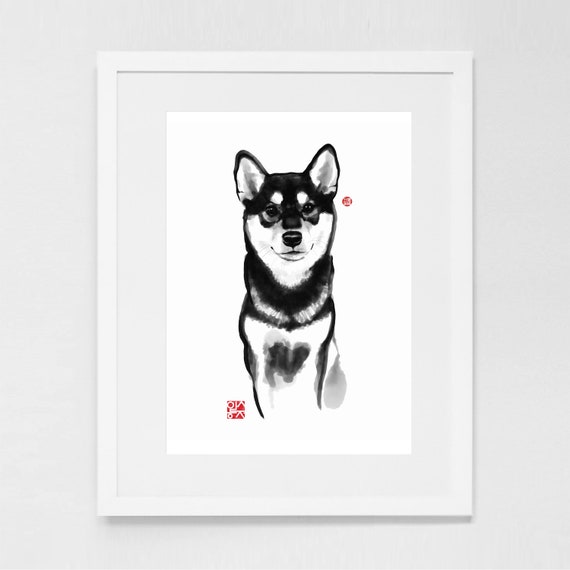The framed watercolor picture features a black and white husky dog sitting and facing forward, with its pointed ears alert and its mouth closed. The dog's eyes look directly ahead, and it possesses distinct black and white markings with gray blobs particularly noticeable on its tummy. The painting is centered within a rectangular, light gray frame hanging on a matching light gray wall. In the bottom left corner of the artwork, there's a red box with white lettering, likely the artist's signature or watermark. Additionally, there is a subtle red bubble in the upper right quadrant of the image. The overall style of the painting resembles a sketch with a white background, emphasizing the delicate yet vivid watercolor technique used by the artist.